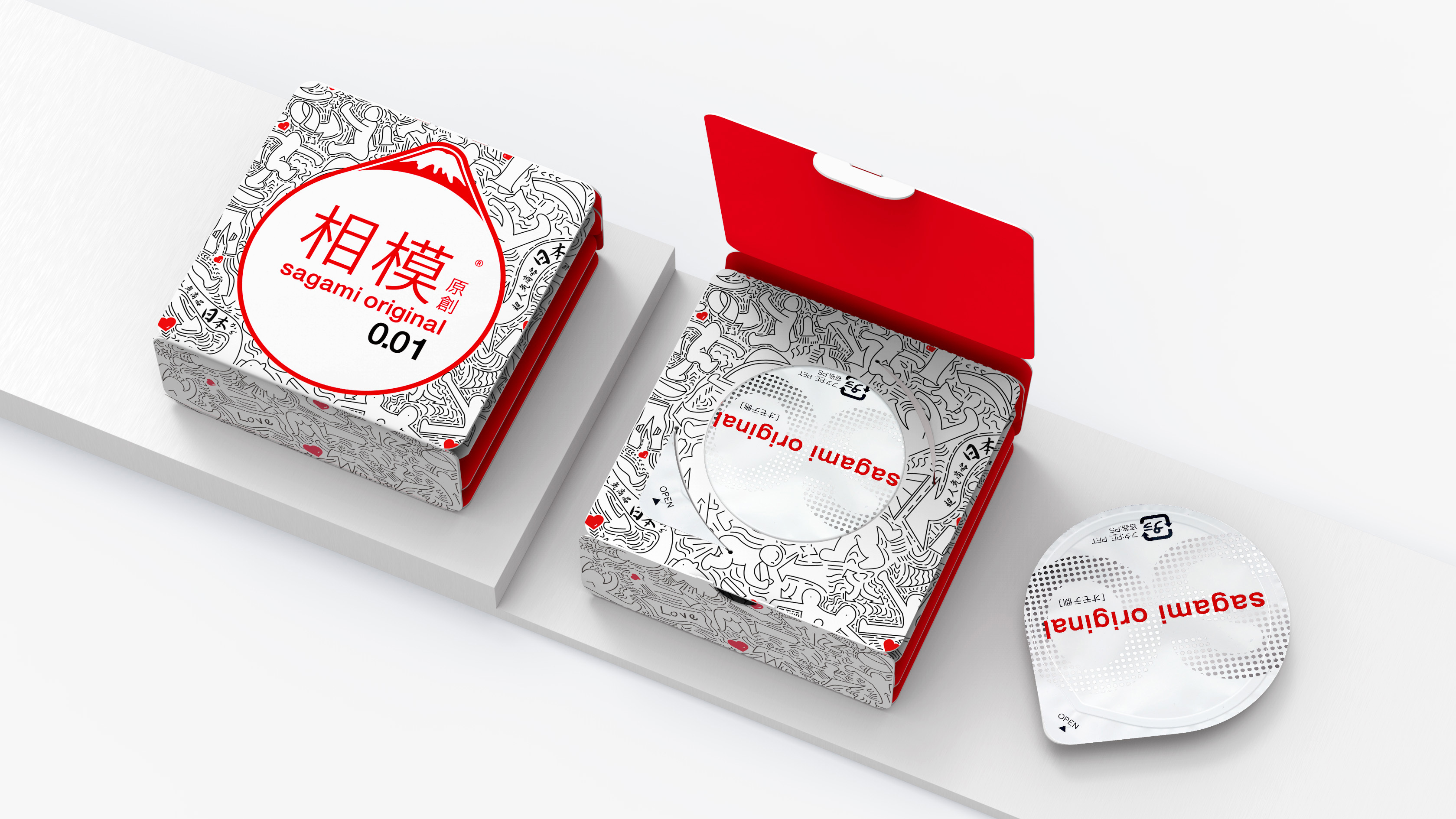The image features three distinct stages of the Sagami Original 0.01 product displayed on a white surface against a white background. On the left, there is a closed box elevated slightly on a ledge, adorned with red sides, red text, and a white circle outlined in red. This circle features Asian characters above the product name "Sagami Original" in red, and "0.01" in black. The box in the center is partially open, revealing a red interior flap and the same design elements as the closed box. To the right, the product itself is shown outside the box, appearing as a circular pouch with a small knob at the bottom. The pouch mirrors the box's design, displaying "Sagami Original" and associated markings in the same color scheme. The entire arrangement is set on a slightly angled surface, with the left side marginally higher due to the ledge.